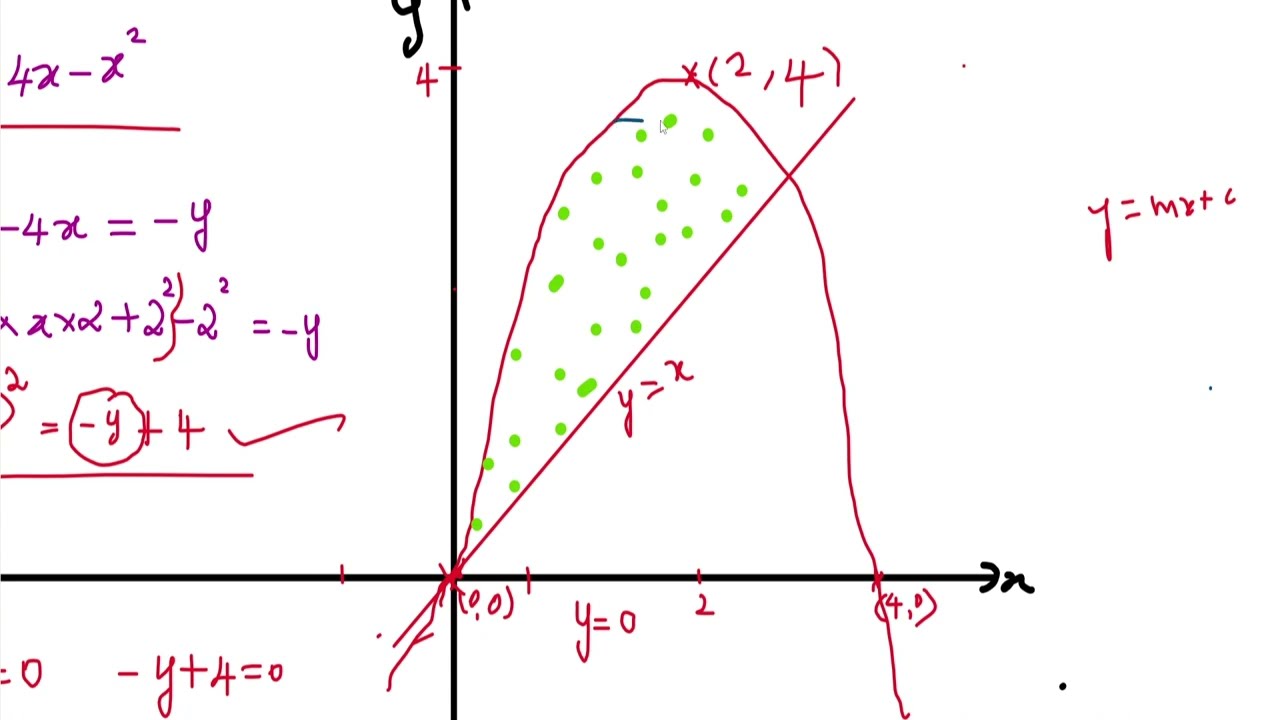The image is a detailed mathematical graph on a horizontal whiteboard, potentially from a math class, featuring both algebra and calculus elements. Dominating the graph are the x- and y-axes drawn in thick black lines, clearly labeled with corresponding coordinates. A distinctive red straight line, labeled "y = x," bisects the graph, intersecting both the axes and a conspicuous bell-shaped curve, reminiscent of a mountain, which crests at the y-axis point labeled "4" before descending and crossing the x-axis at "4,0." 

The area enclosed between this curve and the straight line is filled with numerous green dots, appearing to be around 26-27 in total. The graph also includes multiple equations written in various colors (red, purple, black, and blue) scattered predominantly in the upper left corner and along the graph, although some of these equations are truncated and partially obscured by the frame of the image. Key equations visible include "4x - x²," "negative 4x = -y," and segments of others like "2x something plus 2²," and "negative y + 4 = 0," which also appears underlined with a check mark. Written in red, the equation "y = mx + 6" is visible on the far right side of the graph. The chaotic yet structured distribution of dots and lines along with the varied equations contributes to the intricate tapestry of mathematical relationships being depicted.